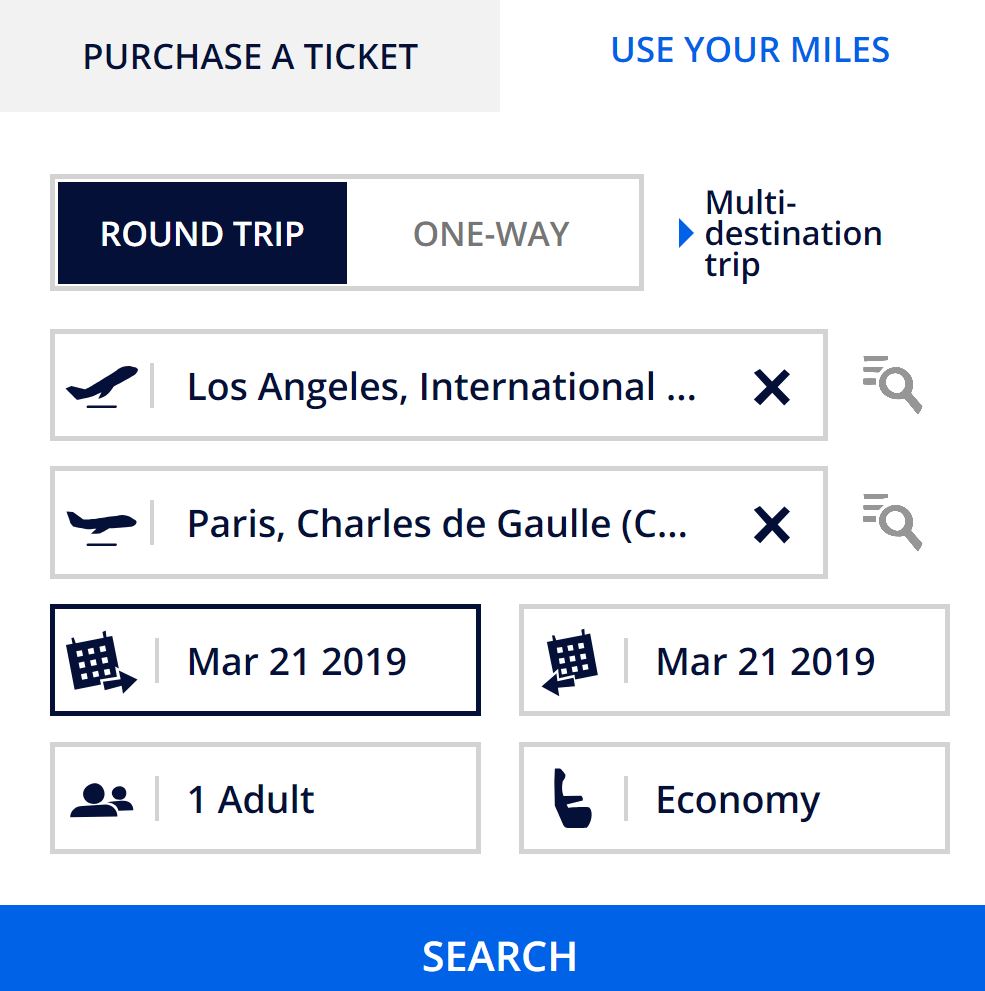Screenshot of a flight booking interface showing a user purchasing a ticket. The interface is rectangular with a predominantly white background. At the top, a gray section with dark blue text reads "Purchasing Ticket." To the right, a white section with royal blue text offers an option to "Use Your Miles." Below this, there is an area for selecting the trip type: round trip, one way, or multi-destination. The selected option is a round trip from Los Angeles International Airport (LAX) to Paris Charles de Gaulle Airport (CDG) dated March 21st, 2019, for one adult in economy class. A conspicuous search bar, highlighted in bright royal blue, allows users to proceed with the booking.